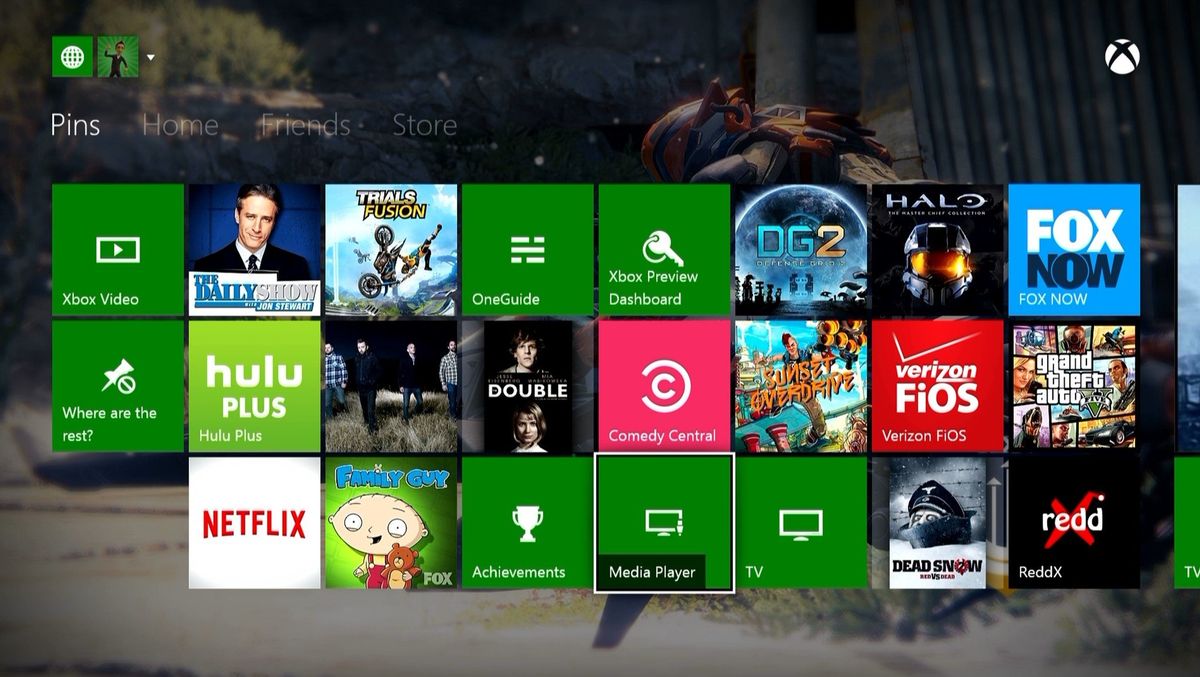This image displays the Xbox home screen, likely captured from a laptop or TV. In the top left corner, a green square features a clear white globe icon. Adjacent is another green square containing a profile avatar, which appears to be male. On the top right, the iconic white Xbox logo is visible. Below, on the left side, the navigation menu highlights "Pens," with options for "Home," "Friends," and "Store" beneath it. 

The main display is organized into three rows of app icons. The first row includes: Xbox Video, The Daily Show, Trials Fusion, OneGuide, Xbox Preview, Dashboard, DG2, Halo, and Fox Now. The second row features apps including Hulu Plus and one displaying an image of four gentlemen, followed by icons for Double, Comedy Central, and Sunset Overdrive, continuing to the screen's end. The third row concludes with a notable red icon overlapping an 'X.'